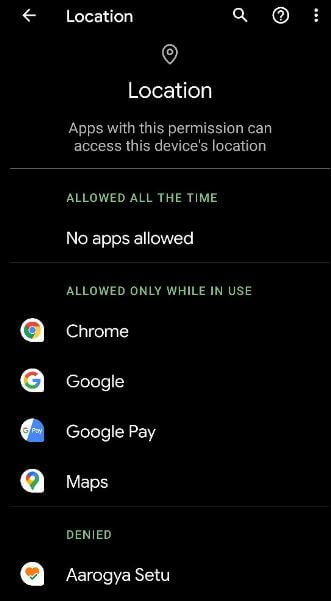Screenshot Description:

The screenshot features a predominantly black background with white and other colored text elements, designed for a user interface displaying location settings. 

In the top left corner, there is a white arrow pointing to the left, adjacent to the word "Location" in white font. 

In the top right corner, three white icons are visible: a magnifying glass, a circle with a question mark inside, and three vertical dots representing a menu drop-down.

Central to the image, slightly below the middle, is a prominent teardrop shape with a circle inside it, symbolizing location. Beneath this icon, "Location" is written in bold white font. Further down, in smaller gray font, it states: "Apps with this permission can access this device's location." 

A white horizontal line divides this section from the following information. Below the line, in light greenish, all capital letters, it reads: "ALLOWED ALL THE TIME," followed by the note "No apps allowed" in bold white font.

Another white horizontal line splits the next section. Below this, it says "ALLOWED ONLY WHILE IN USE," followed by a list of apps each with their corresponding icons:
- Chrome: red, green, and yellow circle with a blue center
- Google: Google’s multicolored G logo
- Google Play: Google's triangular Play Store icon
- Maps: Google Maps' multicolored location pin icon

A dividing line follows this list, leading to the final section labeled "DENIED" in bold white font. Beneath it, "Aragoya C2" is listed without an icon.

The layout is symmetrical, with a clean visual hierarchy making it easy to distinguish between different permission states and their associated applications.